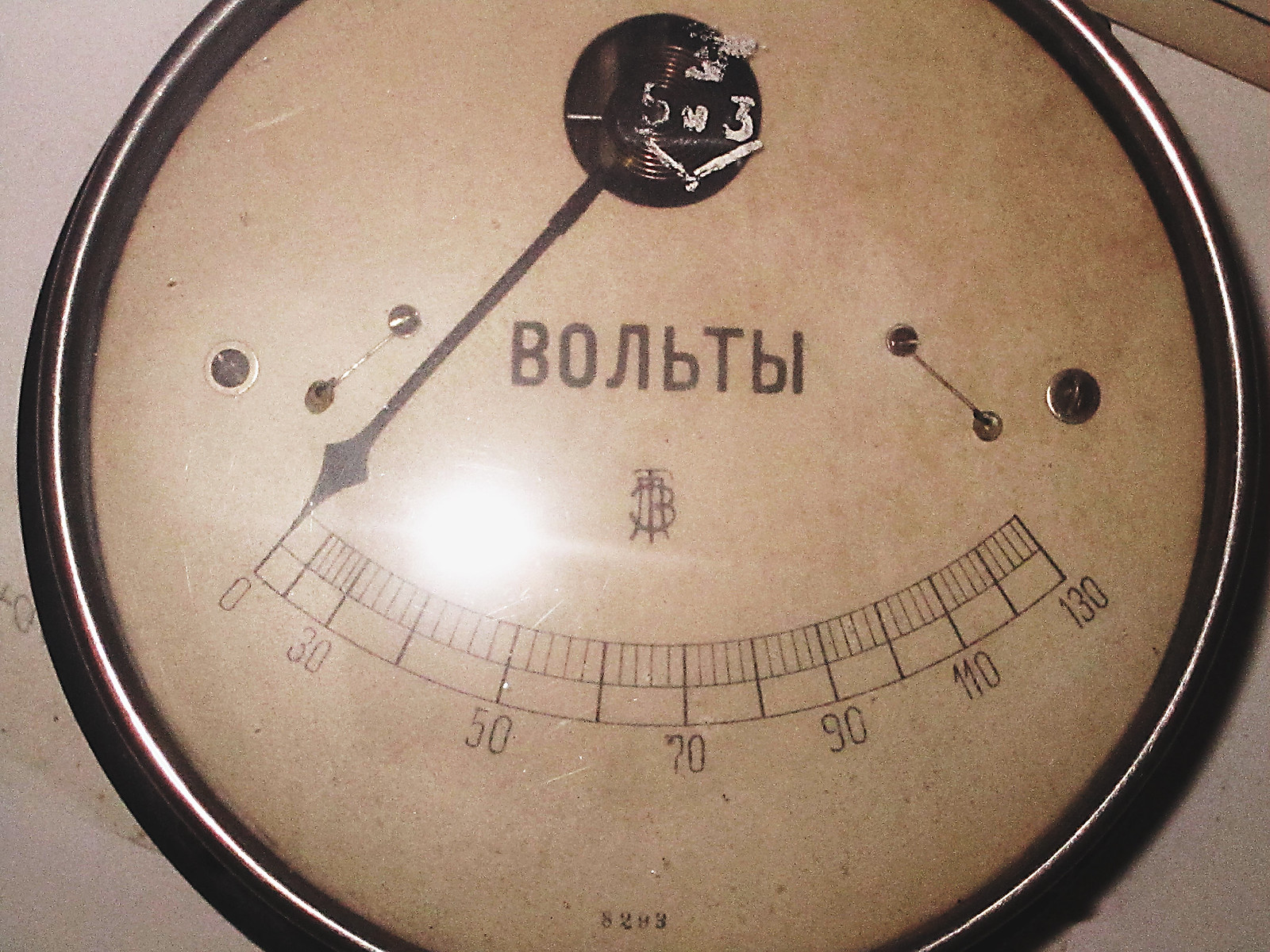This is a color photograph featuring a close-up view of a measuring device, resembling a scale or odometer. Dominating the central part of the image is a circular gauge with a thin black needle pointing to a measurement. The top section of the gauge displays white numerals, including a '5' and a '3', on a black background. Surrounding the needle and the numerals are some unidentified letters that appear to be in a non-English script. Below these letters, the scale is marked with numbers incrementing from 0 to 130 in irregular intervals: from 0 to 30 in smaller increments, and then continuing with larger gaps to 50, 70, 90, 110, and finally 130. At the very bottom of the gauge, a small digital display reads '8293'. There is a noticeable glare of light reflecting off the left side of the gauge, adding a touch of brightness to the otherwise muted, tan-colored background.